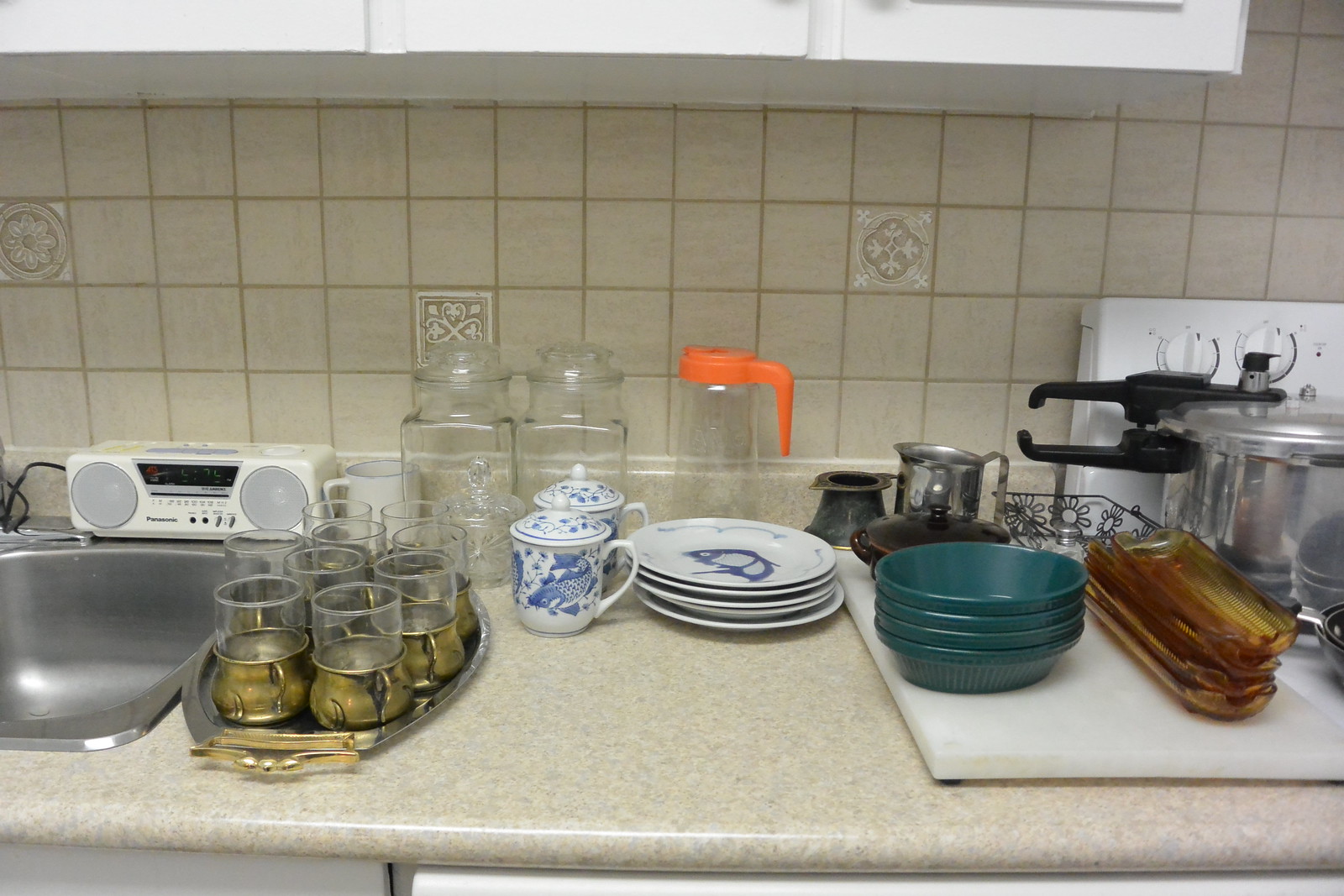The image depicts a kitchen countertop adorned with various items and detailed elements that highlight its design and functionality. The countertop itself is made of laminate, exhibiting a whitish-brown hue with a predominance of white. The backsplash, crafted from nude-colored tiles, features an intricate pattern of grey-colored mortar separating the individual squares. Amidst the uniform tiles, there are intermittent decorative tiles showcasing unique designs, including a snowflake, hearts, and a flower within a circle.

On the countertop, a collection of kitchenware is neatly arranged. There are stacks of white plates with blue patterns, alongside turquoise bowls that add a pop of color to the scene. An old-timey Panasonic boombox from the 1980s with a digital clock is present, flanked by speakers on either end, providing a nostalgic touch. Additionally, several clear glass canisters are lined up against the backsplash, though they appear to be empty, contributing to the organized yet sparse aesthetic of the kitchen setting.